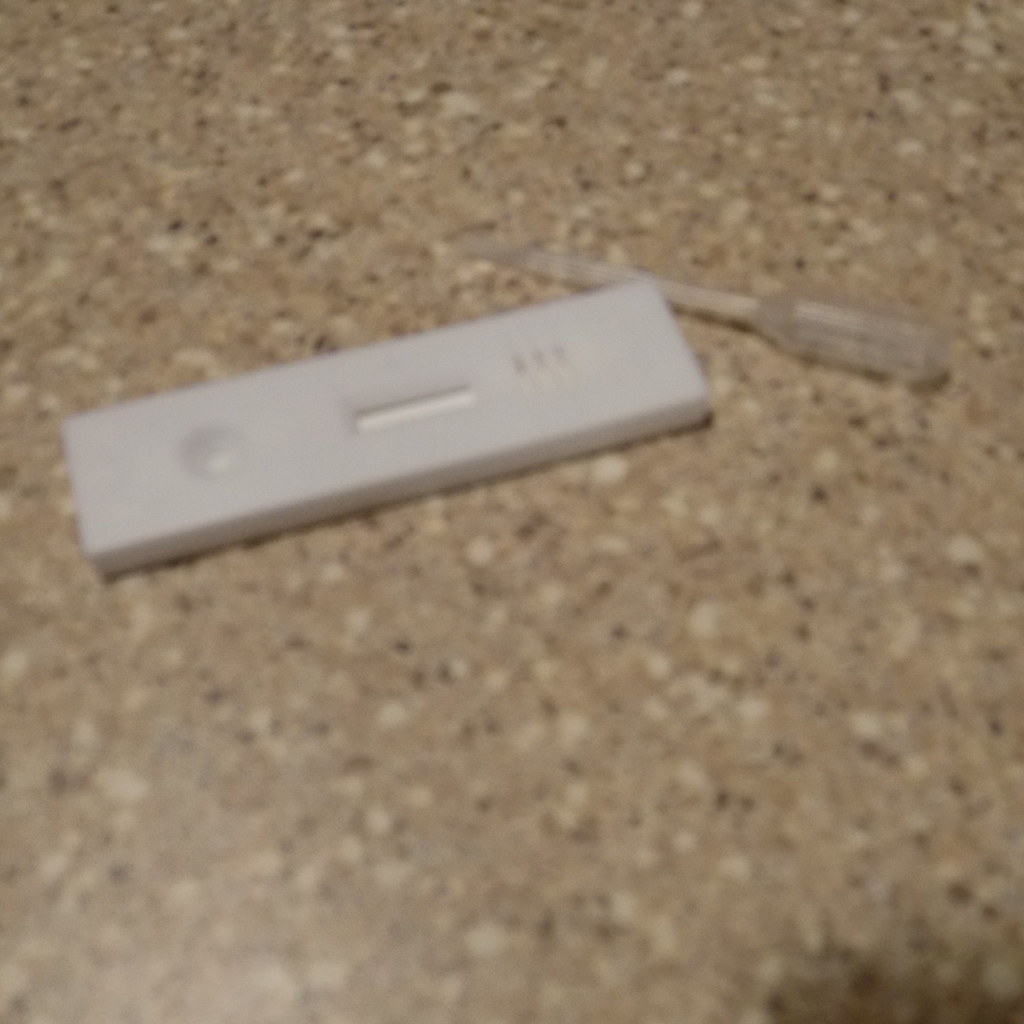A slightly blurry photograph captures a speckled countertop featuring an intricate blend of tan, white, black, and brown colors. The countertop's surface exhibits a distinct pattern, accented with white flares and portions that appear washed out. Shadows cast upon the countertop add depth to the scene. Central to the image is a rectangular white object resting on the surface, distinguished by a white dash in its middle, three white line dashes near the bottom, and a circular white dash at the top. Off to the side, a clear plastic object is visible, consisting of a thicker handle and a slim body. No other objects are present in the photograph. The grainy texture suggests that this image may have been taken some time ago, lending it an older, somewhat vintage appearance.